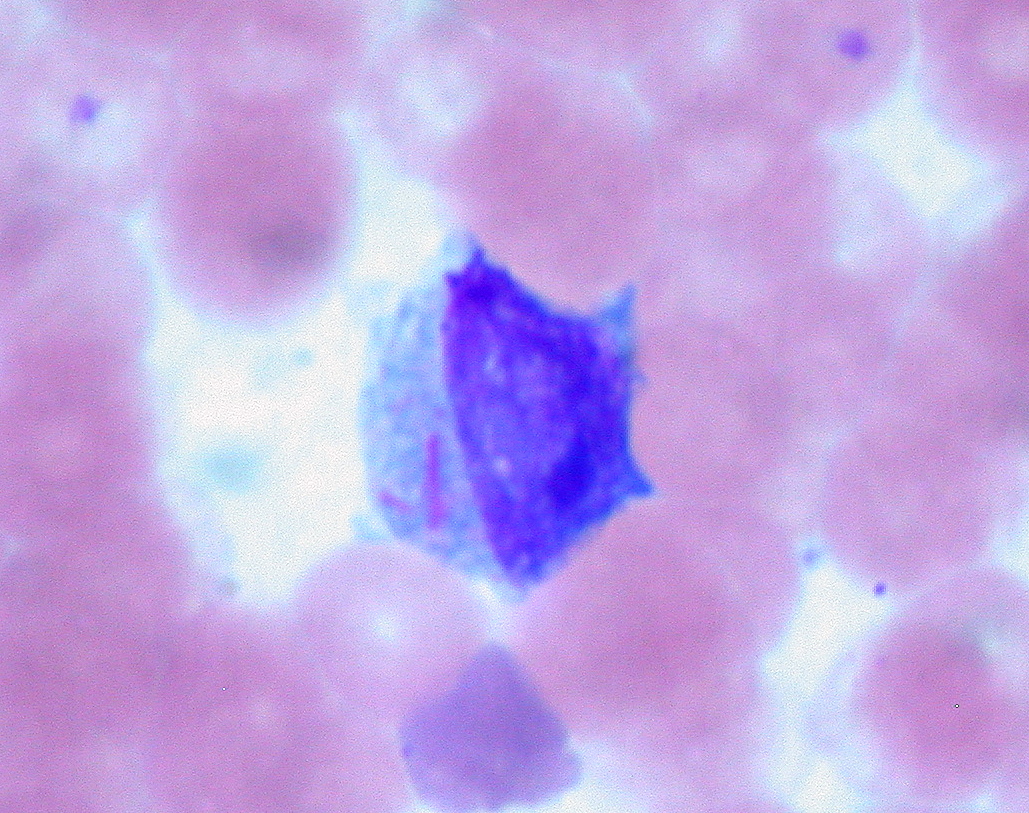The image features an intricate, colorful scene that resembles a high-resolution microscopic view or a piece of abstract art. At the heart of the composition is a near-perfect circle divided down the middle; the left hemisphere is a pale blue, while the right is a vivid dark blue. Amidst this central feature, a darker purple sphere stands out prominently. Surrounding the central circle are numerous pale pink, cotton ball-like structures, which could be described as puffs or globes. Interspersed within are purple specks and some cells with red and purple dots, suggesting a cellular or molecular nature. A striking bright white area pierces through the scene, adding vibrancy and depth. There are no identifiable text or labels, leaving the interpretation open to scientific or artistic perspectives.